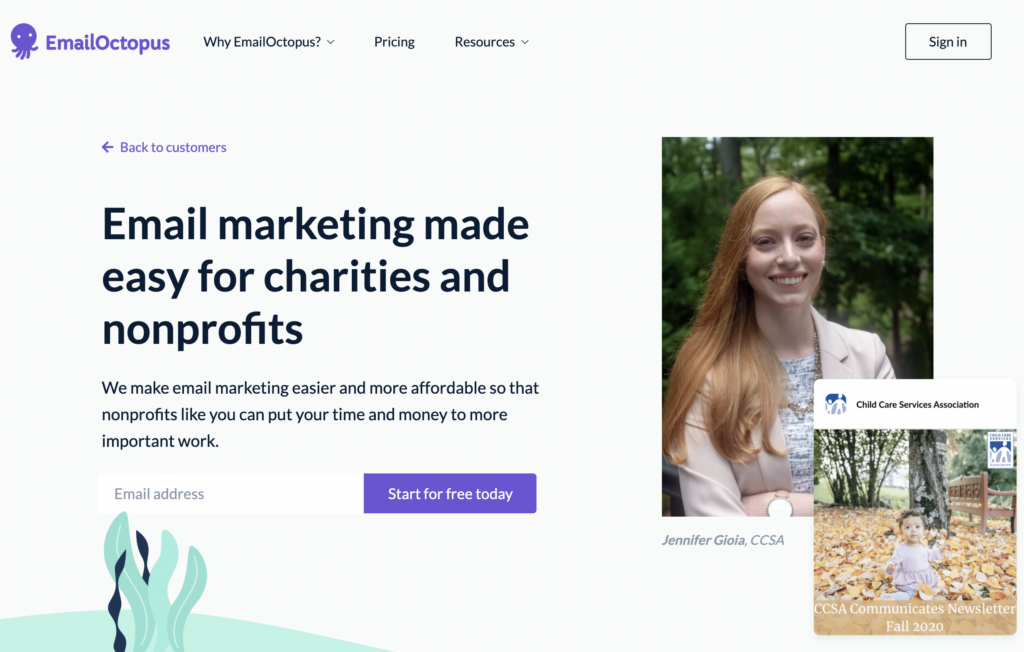The image features the homepage of the website "Email Octopus." At the top, the site's name "Email Octopus" is displayed in purple, written as a single word. The navigation menu includes sections like "Why Email Octopus?", "Pricing," and "Resources." Towards the right side of the header, there is a sign-in box for returning users.

A prominent purple arrow points backward with the text "Back to Customers," also in purple. The main headline reads, "Email marketing made easy for charities and nonprofits." This is followed by a subheading that states, "We make email marketing easier and more affordable so that nonprofits like you can put your time and money to more important work."

Below this text, there is a box inviting users to enter their email address and sign up to "start for free today," with the phrases "start for free today," "Back to Customers," and "Email Octopus" highlighted in purple for emphasis.

At the bottom of the screen, there is a graphic, likely the website's logo, though it is not clearly visible. On the right-hand side of the page, two overlapping pictures are displayed. The larger, top picture features a young, pretty woman with long red hair, wearing a business jacket and folding her arms. The image is captioned with her name, "Jennifer Giola," and her title, "CCSA."

Overlapping the bottom right corner of Jennifer's picture is a smaller image belonging to "Child Care Services Association." This smaller image shows a baby lying among autumn leaves and serves as an advertisement for the organization's fall 2020 newsletter.